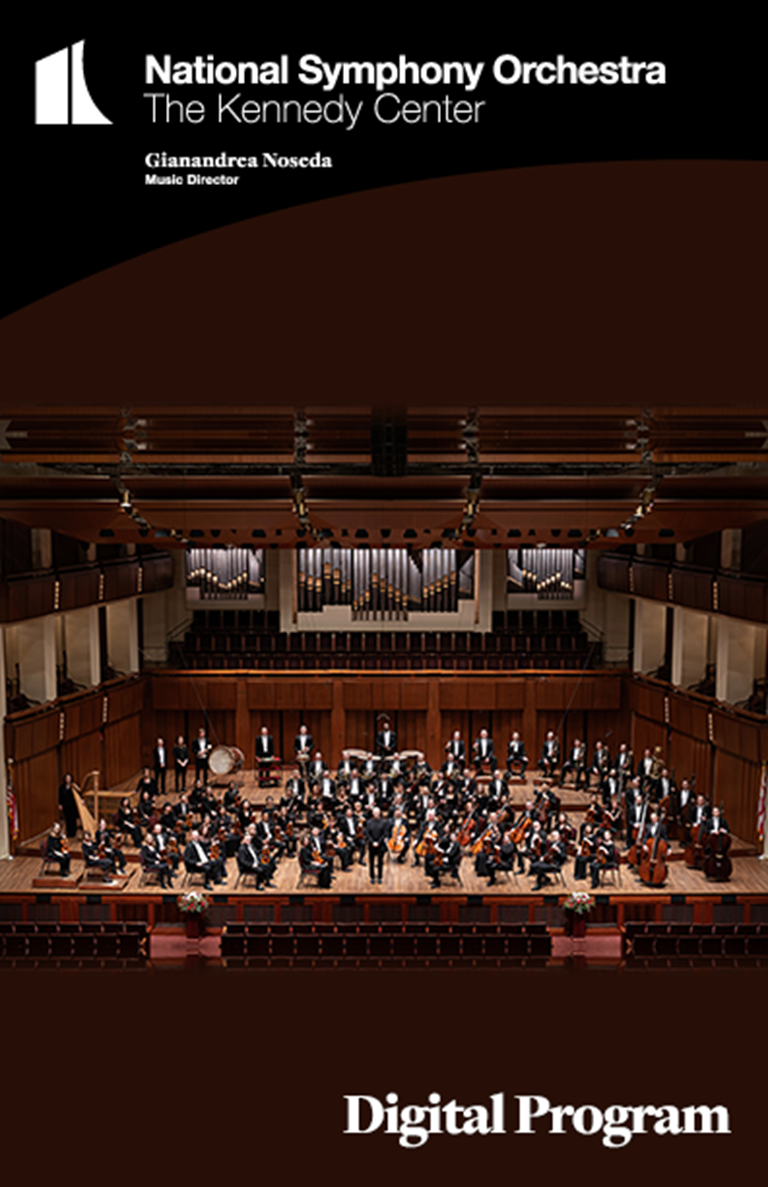The advertisement showcases a captivating image of the National Symphony Orchestra performing at the Kennedy Center under the direction of Guy Andria Nozada. The photograph, rectangular with the shorter edge horizontal, captures the grandeur of the venue from a balcony viewpoint, emphasizing the full orchestra set on the stage below. At the top of the image, the text reads "National Symphony Orchestra, The Kennedy Center, Guy Andria Nozada, Musical Director." Dominating the center is the orchestra, positioned meticulously with every instrument visible, ranging from drums to cellos and basses. The players, captured from a distance, appear smaller, allowing the entirety of the symphony and their setting to be seen. The stage is flanked by two large potted plants at the extreme left and right edges, adding a touch of greenery to the elegant scene. At the bottom right corner, the words "Digital Program" are displayed, indicating a modern, perhaps virtual, offering of the performance.